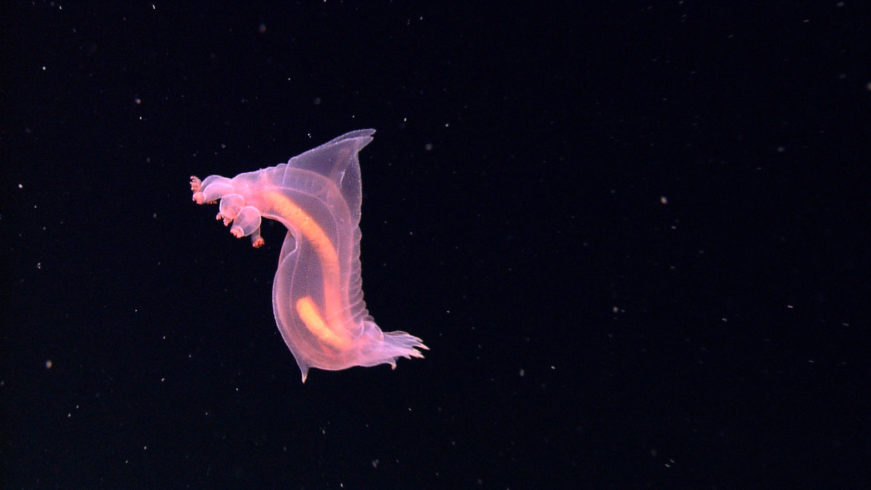The image captures a mysterious underwater or microscopic creature against a pitch-black backdrop sprinkled with white flecks that resemble stars. The creature, which is pinkish-purple, appears translucent, allowing a clear view of its internal orange tube-like organ, possibly an intestine, curling inside its body. The organism resembles a chubby caterpillar or a microscopic animal seen under high magnification. It has a distinct head adorned with several short, tentacle-like growths ending in small orange knobs. Its body features delicate, translucent fins and tails, giving it an otherworldly appearance as it floats in its dark, liquid environment. The image intriguingly blurs the lines between an oceanic scene and a microcosmic view, making the creature look both alien and familiar.